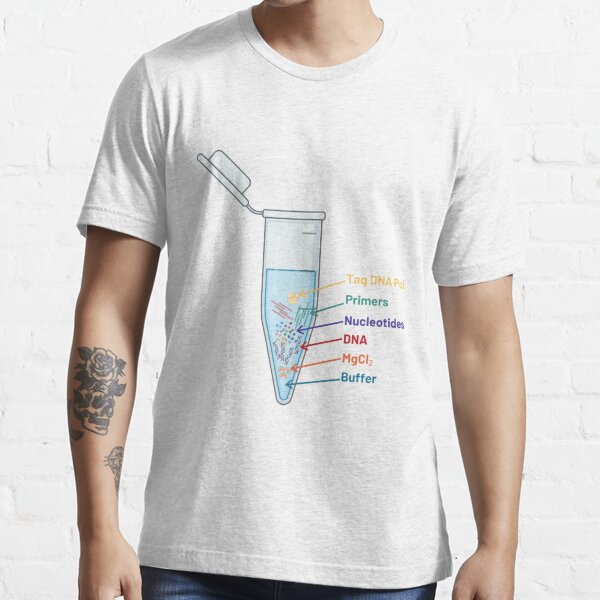The image features a young Caucasian man, primarily visible from the waist up, positioned against a barely discernible white center-block wall that enhances the overall brightness and focus on him. He is dressed in a white t-shirt adorned with a detailed, colorful illustration of a chemistry flask. Inside the flask, a blue liquid labeled as "buffer" is depicted, with various other components like "tagged DNA pool," "primers," "nucleotides," "DNA," and "MgCl2" enumerated in different colors, creating a vibrant, science-themed design. Additionally, the man has a noticeable black tattoo of a rose with surrounding leaves on his right forearm, along with the edge of another, indeterminate tattoo. His attire is completed with blue jeans, but only the top of the jeans is visible as the image cuts off at his chin, showing just a hint of his facial features. The scene and lighting suggest the image might be intended for advertising the t-shirt, likely appealing to fans of chemistry or scientific themes.